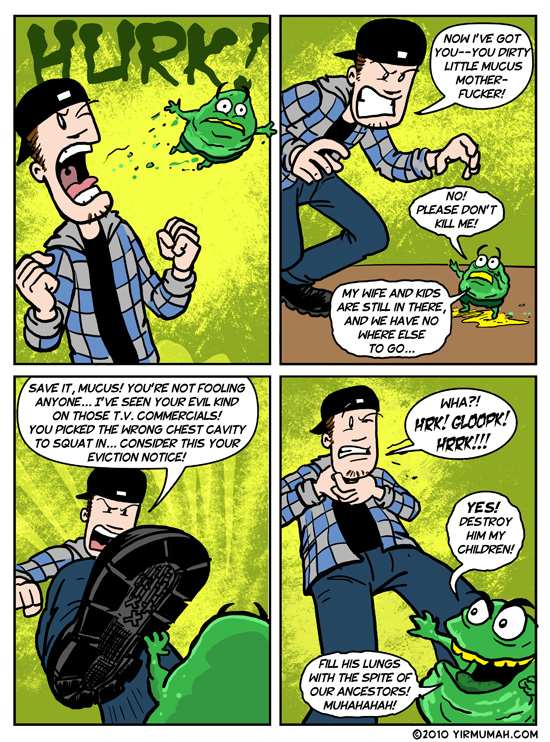The image is a four-panel comic strip predominantly in shades of green, black, and gray. The comic features a white male wearing a blue and gray checkered hooded sweatshirt over a black t-shirt and a black hat. The background is mostly green, with the mucus character being bright green with white eyes.

In the first panel, the man is shown with his mouth wide open, screaming "HURK!" at the green mucus-like character. The man appears very angry and intense. 

In the second panel, the man is bent over, looking disgruntled. A speech bubble next to him reads, "Now I've got you, you dirty little mucus motherfucker." The green mucus character responds with, "No, please don't kill me. My wife and kids are still in there, and we have nowhere else to go."

In the third panel, the man is about to stomp on the mucus character and exclaims, "Save it, mucus! You're not fooling anyone. I've seen your evil kind on those TV commercials. You picked the wrong chest cavity to squat in. Consider this your eviction notice."

In the fourth and final panel, the man is holding his throat, while the mucus character, now seemingly gaining the upper hand, says, "Yes, destroy him, my children! Fill his lungs with the spite of our ancestors."

Throughout the panels, the comic maintains a humorous yet slightly grotesque tone, with exaggerated expressions and dramatic dialogue, characteristic of a cartoon strip one might find in a newspaper or magazine.